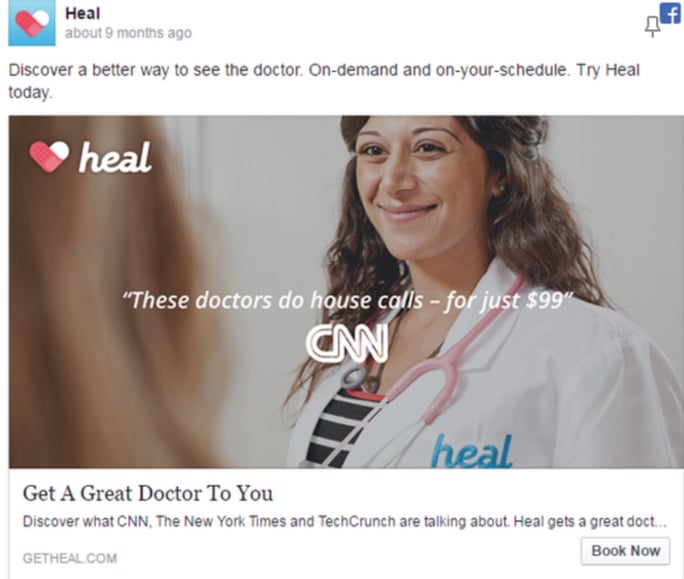This image appears to be an advertisement for a healthcare service called "Heel." The top two inches feature a white border with a blue square in the top left corner that contains a heart logo; the heart is predominantly red with a white upper right corner. Adjacent to this is the word "heel" in bold black letters. Below are the words "about nine months ago" in gray, alongside a small pin icon and the Facebook icon.

To the left, in black lettering, the ad reads: "Discover a better way to see the doctor. On-demand and on-your-schedule. Try Heel today."

The main focus of the image is a smiling woman with brown eyes and long brown hair. She is wearing a black and white striped shirt under a doctor's coat adorned with the "Heel" logo in teal. A pink stethoscope hangs around her neck. Behind her is a white wall; to the left, the back of another woman's head with blonde hair is visible. 

In the top left corner, there's a red heart logo with a small white section. To its right, in bold white letters, the word "heel" is displayed. Across the woman's neck, in white text within parentheses, it reads: "These doctors do house calls - for just $99," and in bold white letters below this, "CNN."

Under the picture on the left side, in large black letters, it states: "Get a great doctor to you." Beneath this, in smaller black letters, it says: "Discover what CNN, The New York Times, and TechCrunch are talking about. Heel gets a great doctor to you."

At the bottom left corner, there is a white tab with a black border that reads "Book now." Below that, in all capital letters and black text, it says "GETHEEL.COM."